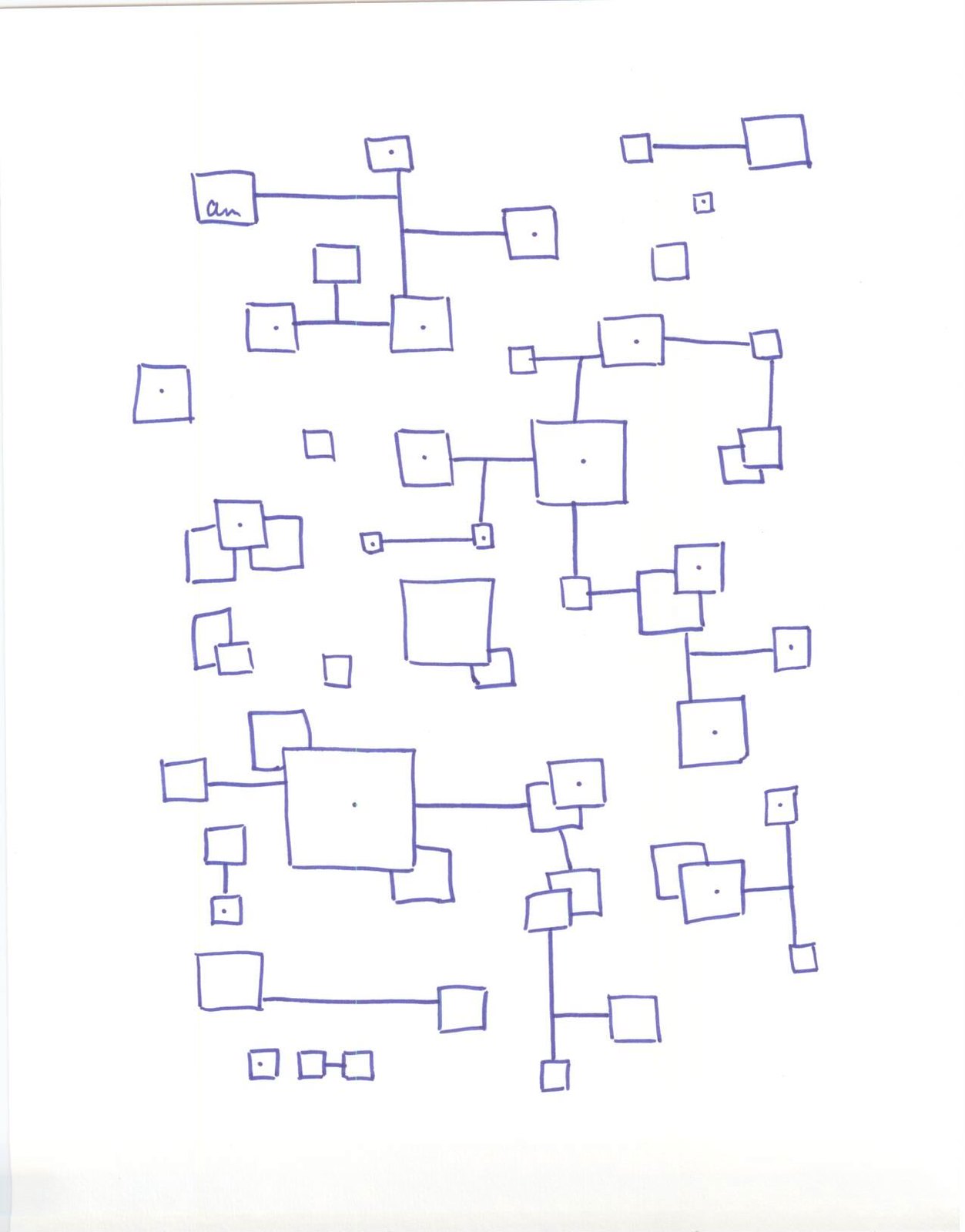This intricate drawing features a complex array of intersecting squares, each intriguingly distinct in its connectivity. While some squares stand alone, others branch out similar to the structure of a family tree—one box dips down and then extends outward to form additional connections. Dots adorn some of these boxes, adding a further layer of detail. Notably, the intersections of the squares are cleverly rendered, with one square always overlapping the other, effectively hiding any underlying lines. This creates a seamless, woven appearance.

The entire illustration is rendered in a blue tone, evoking a maze-like composition of interconnected boxes and lines. Despite the apparent randomness, the drawing maintains a consistent theme: the boxes are exclusively squares, not rectangles. An intriguing feature resides in the top-leftmost square, which appears to contain the beginning of a script, possibly the letters "A N." This adds an element of mystery and invites viewers to ponder the hidden meanings within this captivating, abstract piece.